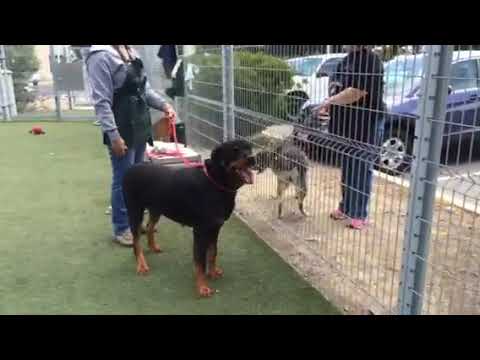In this outdoor image with a black border on the top and bottom, we see two dogs and their handlers separated by a diagonal metal fence. On the left side, standing on a surface that looks like fake green turf, is a Rottweiler with brown and black fur, wearing a pink collar and leash held by a person whose head is cropped out of the picture. This person is clothed in a gray and black long-sleeved top, blue jeans, and an apron. To the right of the fence, the ground is light dirt and the handler is wearing a short-sleeved black t-shirt, blue jeans, and pink tennis shoes. This person is holding a dark gray and white dog on a leash. Behind her, there is a bush to her right and a parking area with several vehicles visible.